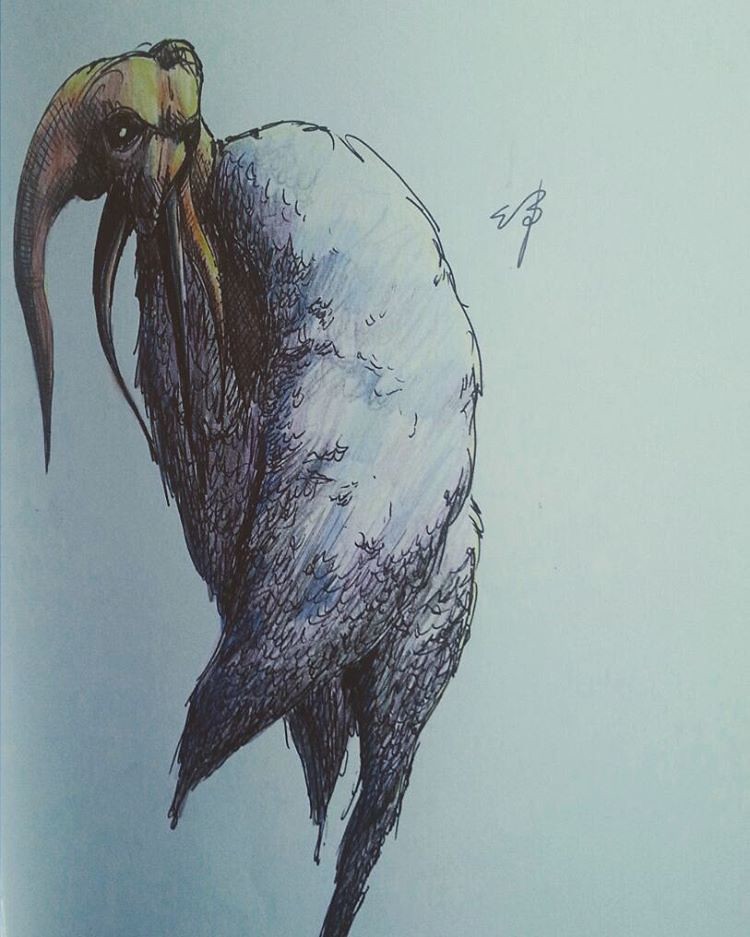This is a detailed drawing of an unusual animal set against a light blue background. The animal's head is prominently featured, facing the viewer with piercing, dark eyes that create a stark contrast against its yellowish complexion. The body of the creature, however, is oriented away from the viewer, adding a sense of curiosity to the composition. The body is large and robust, with distinct legs at the bottom and a tail extending in the opposite direction from the head. The artistic style and unique angle of the subject make this drawing particularly intriguing.